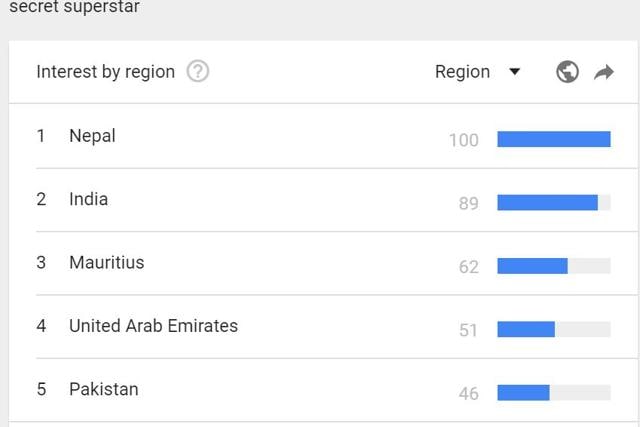This image is a cropped screenshot that unambiguously presents a snippet of data, though it is unclear whether it originates from a website or a software application. The central focus of the screenshot is a table with a clean, white background, delineated by thin, gray lines separating the information into easily distinguishable sections. 

At the top of the image, the title "Secret Superstar" prominently indicates the subject of the data. Below this title, the table is structured with the header "Interest by Region" atop the first column. This header is followed by a list of five regions: Nepal, India, Mauritius, United Arab Emirates, and Pakistan. 

Adjacent to each listed region, a blue bar graph visually represents the percentage level of interest. The lengths of the blue bars vary, with Nepal reaching the maximum at 100%. Following Nepal, the interest levels decrease in descending order: India at 89%, Mauritius at 62%, the United Arab Emirates at 51%, and Pakistan at 46%.

Despite the detailed layout, the screenshot lacks contextual information about what the "interest" pertains to. Therefore, it remains unclear whether these percentages reflect audience interest, search trends, or another metric related to "Secret Superstar."